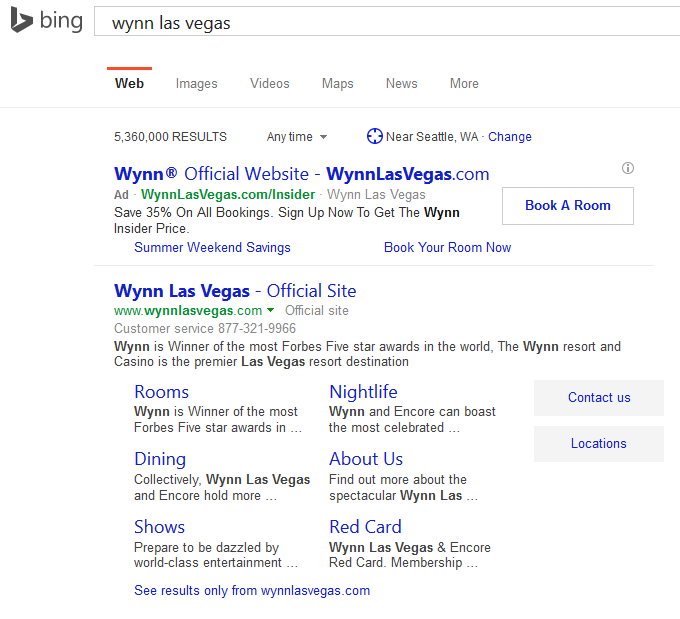**Detailed Caption:**

This image is a screenshot of a Bing web search page. In the upper left corner, the "Bing" logo is displayed in grey alongside a stylized grey 'b' icon. The search bar is a vertical rectangle featuring the query "Win Las Vegas" written in grey font.

Different search categories are listed horizontally below the search bar. An orange vertical line highlights the "Web" category, which is in darker font. Adjacent categories are "Images," "Videos," "Maps," "News," and "More," all in lighter grey font. The search generated approximately 5,360,000 results.

The location setting for the search is near Seattle, Washington, with an option to change the location via a blue clickable link.

At the top of the search results is a sponsored ad for the "Win Official Website" (winlasvegas.com). To the right of this listing, there is a clickable rectangle link that says "Book a Room." The ad notes that you can save 35% on all bookings and encourages users to sign up for the Win Insider price. There are additional clickable links, such as "Summer Weekend Savings" and "Book Your Room Now," both in blue.

The next search result is again for the "Win Official Website," with the URL displayed in green. This listing includes a customer service number and various options you can click within the Win Las Vegas website. The clickable links are arranged in two columns of three links each, in blue font. To the right, there are "Contact" and "Location" links, making the layout symmetrical and straightforward.